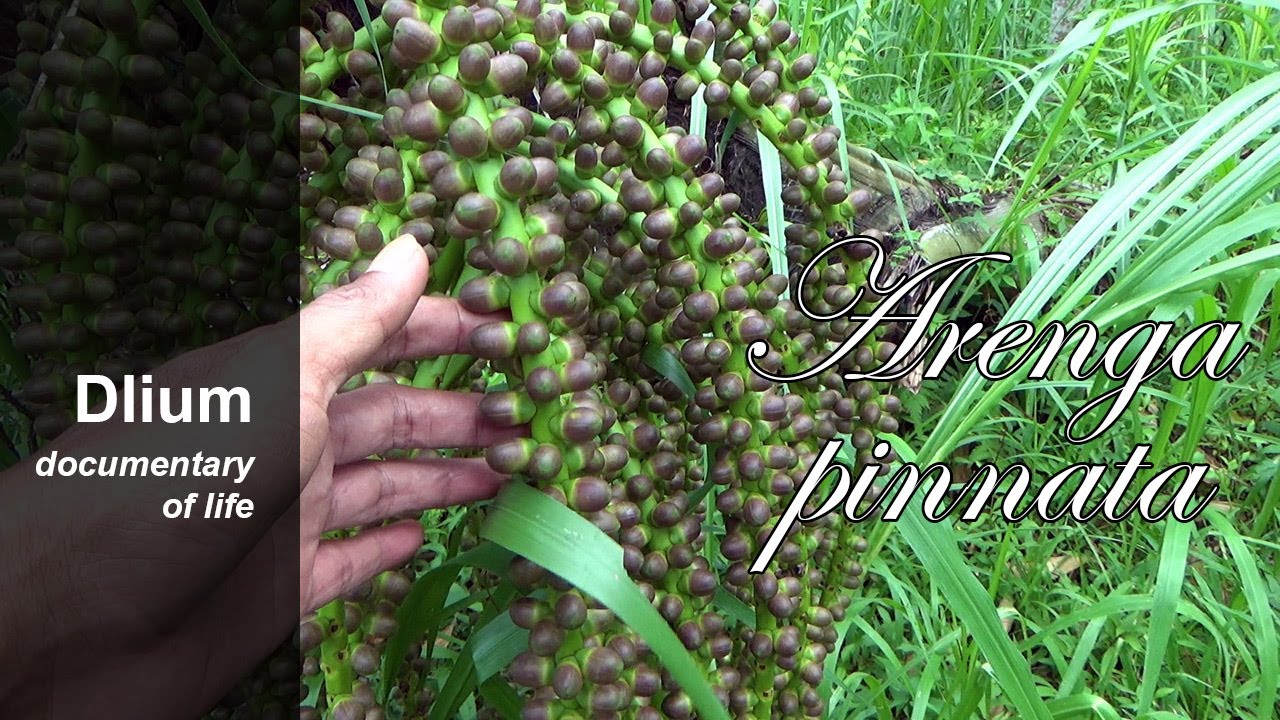In the outdoor image, a semi-transparent, shadowed section on the left is overlaid with white text that reads "Dillium" and "Documentary of Life." A hand enters the frame from the bottom left and is partially covered by this shadow. The hand, positioned so the thumb faces upward, is depicted in natural light to the right of the shadow, grasping bunches of bulbous, purple-brown berries hanging from green stalks. Behind the hand, numerous green plant leaves form the backdrop. Towards the right side of the image, superimposed on the plant and grasses, is additional white text that reads "Arenga Pinnata."